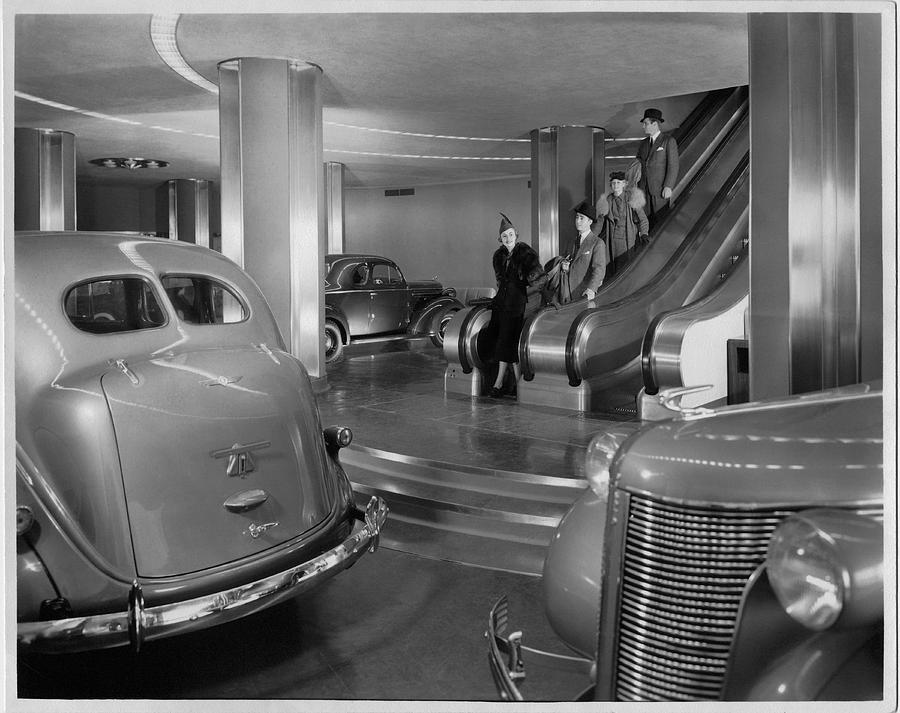This black-and-white photograph, likely taken in the 1940s or perhaps the 1950s, captures a glamorous, high-end setting resembling a luxury hotel parking area or a valet rotunda. The photo features a shiny marble floor with silver-edged steps and two escalators—one going up and one coming down—set amidst silvered columns and well-illuminated ceilings. Four elegantly dressed adults are descending on the down escalator. The first woman wears a chic fur coat and a hat with a feather, followed by a man in a suit holding a raincoat and wearing a fedora. Behind them, another woman in a fur-trimmed coat and hat is accompanied by a second man, also in a dark suit and fedora with a raincoat over his arm. The scene includes vintage, gangster-style luxury cars, such as Mercedes, with only parts of the cars visible—a grille and hood in the right lower foreground and the back of another in the left foreground. The overall atmosphere exudes a feel of sophistication and opulence characteristic of the mid-20th century.